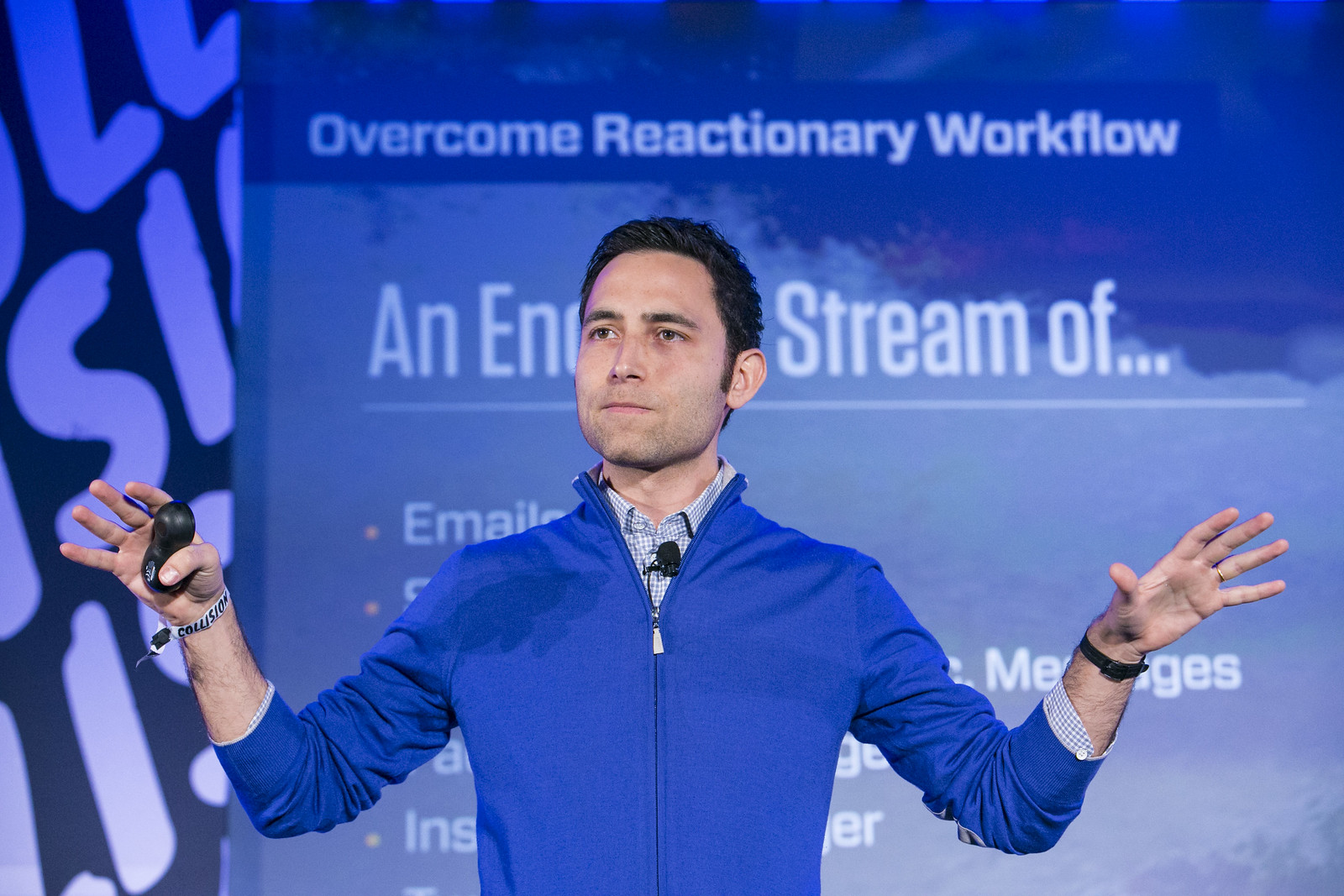A detailed photograph captures a young man, approximately 30 years old, delivering a presentation on stage at what appears to be a professional conference or event. The man, who is not looking directly at the camera, has short black hair and brown eyes. He is dressed in a blue, long-sleeved, zipped-up sweater over a white and blue checkered button-up dress shirt. A small black microphone is pinned to his sweater, indicating he is speaking to an audience. In his right hand, he holds a black presentation clicker, and on the same wrist, he wears a bluish wristband with the word "Collision," which may be related to the event. His left hand is extended outward with fingers slightly spread, adorned with a black bracelet.

The background of the image features a blurred presentation board with partially obscured text due to his position. The legible part of the text reads "overcome reactionary workflow," although the subtitle and bullet points are blocked by his head and upper body. The overall quality of the photo is high, with excellent lighting focusing on the speaker, giving a professional and sharp foreground against a blurred backdrop.